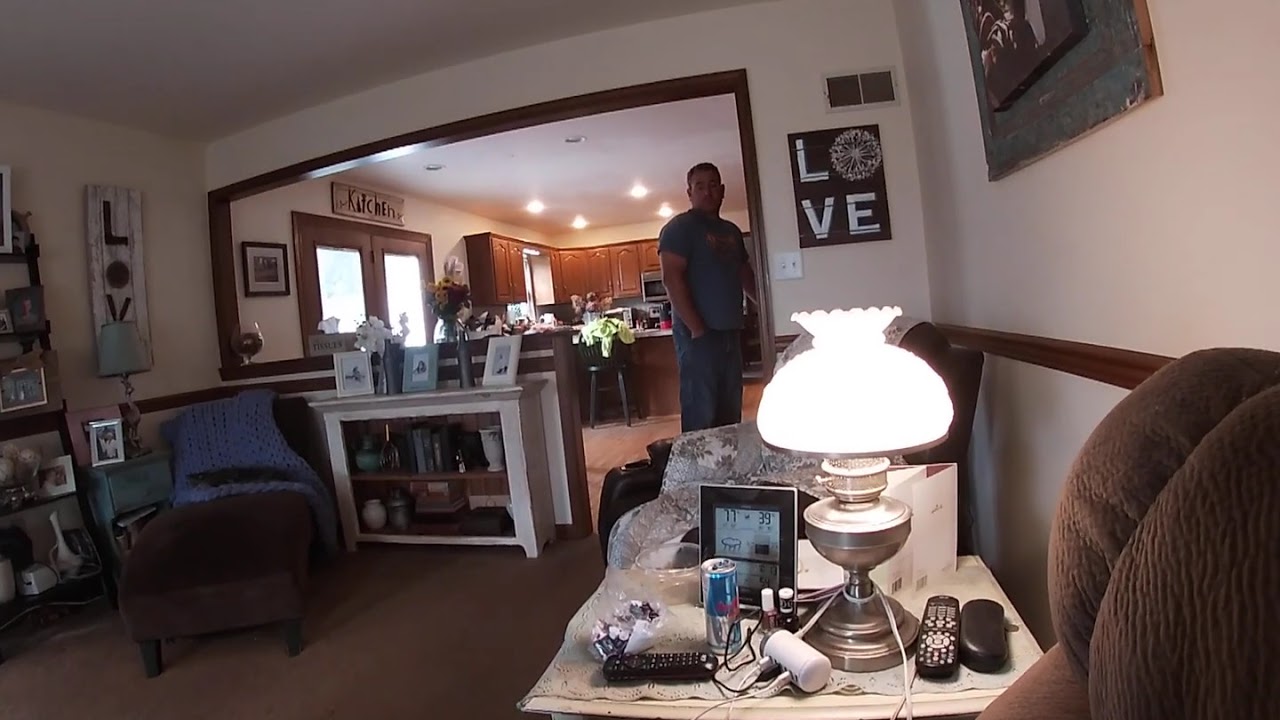In the color photograph of a landscape-oriented interior scene, a man stands in the open doorway of his home, straddling the threshold between the living room and the kitchen. The man, about 40 years old, is dressed in a blue t-shirt and jeans, facing the camera. The living room, depicted as cluttered with various decorations and personal items, features two brown couches—one against the wall under a framed picture—and multiple end tables. 

The foreground includes a small table cluttered with items: a lit gold hurricane lamp, remote controls, a Red Bull can, and an eyeglass case. On the right, a white shelf filled with framed photographs and flowers stands next to a large upholstered brown chair. 

In the background, the more organized kitchen showcases modern elements, with reddish-brown wood cabinets and a microwave. Above the doorway, a small sign reading "L-O-V-E" is affixed to the wall. The scene captures the contrast between the cozy, slightly disordered living space and the cleaner, more streamlined kitchen.